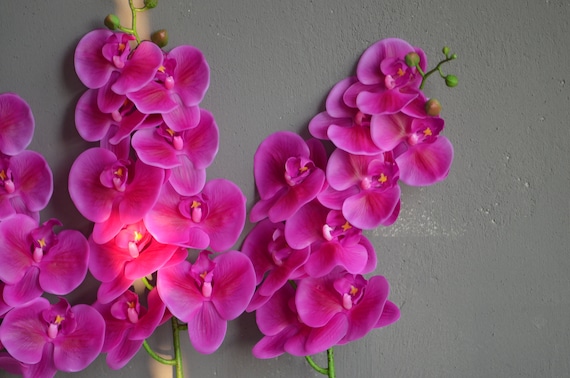The photograph captures a delicate floral arrangement of three vibrant pink-ish orchids set against a worn medium-gray wall. The green stems of the orchids emerge from the bottom of the image, supporting clusters of open, pansy-shaped flowers that gradually transform into buds at the top. Light shines softly on the blooms, highlighting the subtle yellow or pink centers of each flower. The detailed textures of the gray wall, with patches worn to white, contrast beautifully with the bright, natural hues of the orchids, amplified by the gentle overhead lighting, giving the entire setup a serene yet vivid appearance.